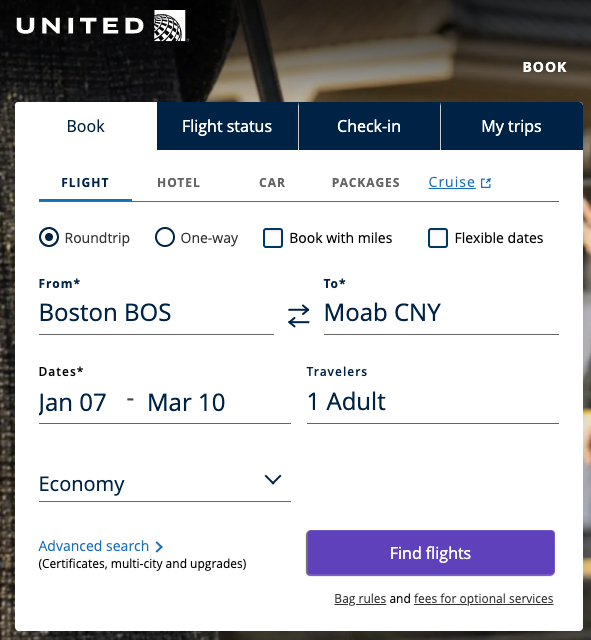On the United Airlines booking webpage, the interface prominently features the United logo in the upper left corner. Adjacent to the logo on the right is a horizontal menu tab titled "Book," which is highlighted in white and uses black font for visibility. 

Below this main menu, there are several navigation tabs, reading "Book," "Flight Status," "Check-In," and "My Trips." The "Book" tab is highlighted with a white background and black text, while the other tabs are dark blue with white font.

In the detailed booking section, the "Flight" tab is distinguished with an underline and highlighted in blue. Other options under this section include "Hotel," "Car," "Packages," and "Cruises," where "Cruises" also stands out with a blue underline, emphasizing its clickable nature.

Within the "Flight" section, the user has selected the "Roundtrip" option, indicated by a tick mark. The departure and arrival details are filled as follows: from Boston (BOS) to MOA (code: CN), with travel dates from January 7th to March 10th. This itinerary is set for one adult in the economy class. An expandable menu allows further customization. 

For more specific searches, there is an "Advanced Search" option in blue, accompanied by a right arrow. Below, additional options include "Certificates," "Multi-city," and "Upgrades," written in black.

At the bottom-right corner of this section, a purple "Find Flights" button with white font invites the user to proceed. Below this button, there are links for "Bag rules" and "Fees and optional services," both underlined, providing additional information to the user.